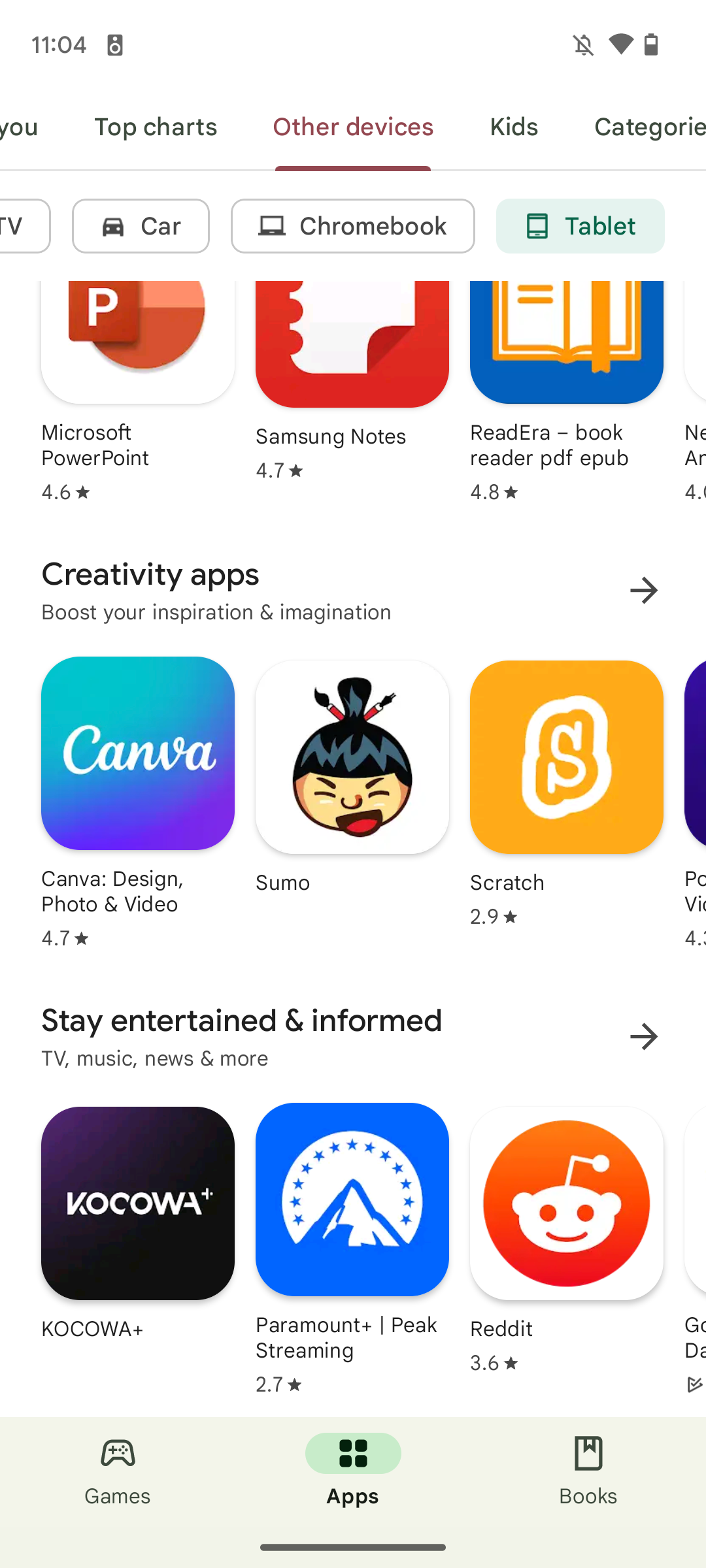In this detailed screenshot of a user's phone on a Google or Android store, several key elements can be observed. Starting from the top right, the battery icon indicates it's half full, with a fully filled Wi-Fi icon just to its left, denoted by a dark gray color. A bell icon with a slash through it is also visible, signifying notifications are muted. On the top left, the time displayed is 11:04, accompanied by a camera icon. 

Just beneath this bar, several navigation options are visible. The central option, "Other Devices," is highlighted in red and underlined. To its left lies the "Top Charts" option, while to its right, "Kids" and "Categories" are displayed. A light gray line separates these navigation choices from the content below.

Below this line, several category boxes are aligned horizontally—"TV" on the far left, followed by "Car," "Chromebook," and "Tablet." Under these categories, a grid of app icons appears, each within its own square frame. Notably, the first app displayed is Microsoft PowerPoint, followed by Samsung Notes, and then Red Era Book.